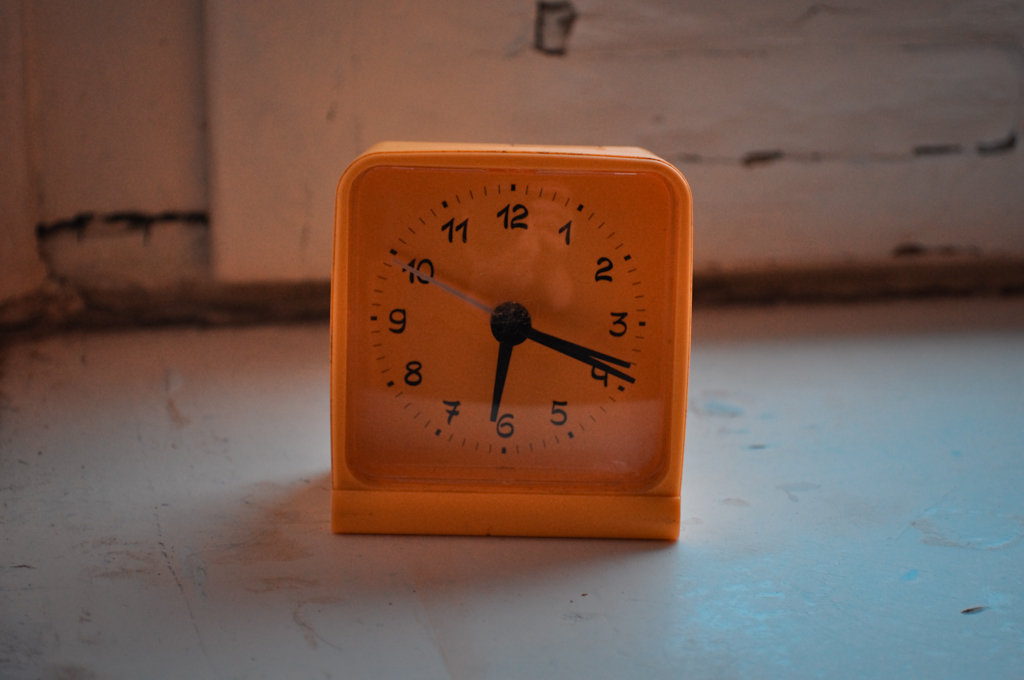The image features a vintage, light orange travel alarm clock with black hour and minute hands and a white second hand. The time displayed is approximately 6:18. The clock rests on a heavily worn and marked surface, which could either be a floor or a table. The background reveals a distressed wall with dark streaks of dirt or wear, and a blackened area resembling rust where the clock meets the wall. The scene has an intriguing and somewhat incongruous vibe, as one might not expect to find a travel alarm clock in such a dilapidated setting. The lighting is minimal, coming from above and casting a faint glow on the back of the clock, adding to the overall starkness and moodiness of the composition.